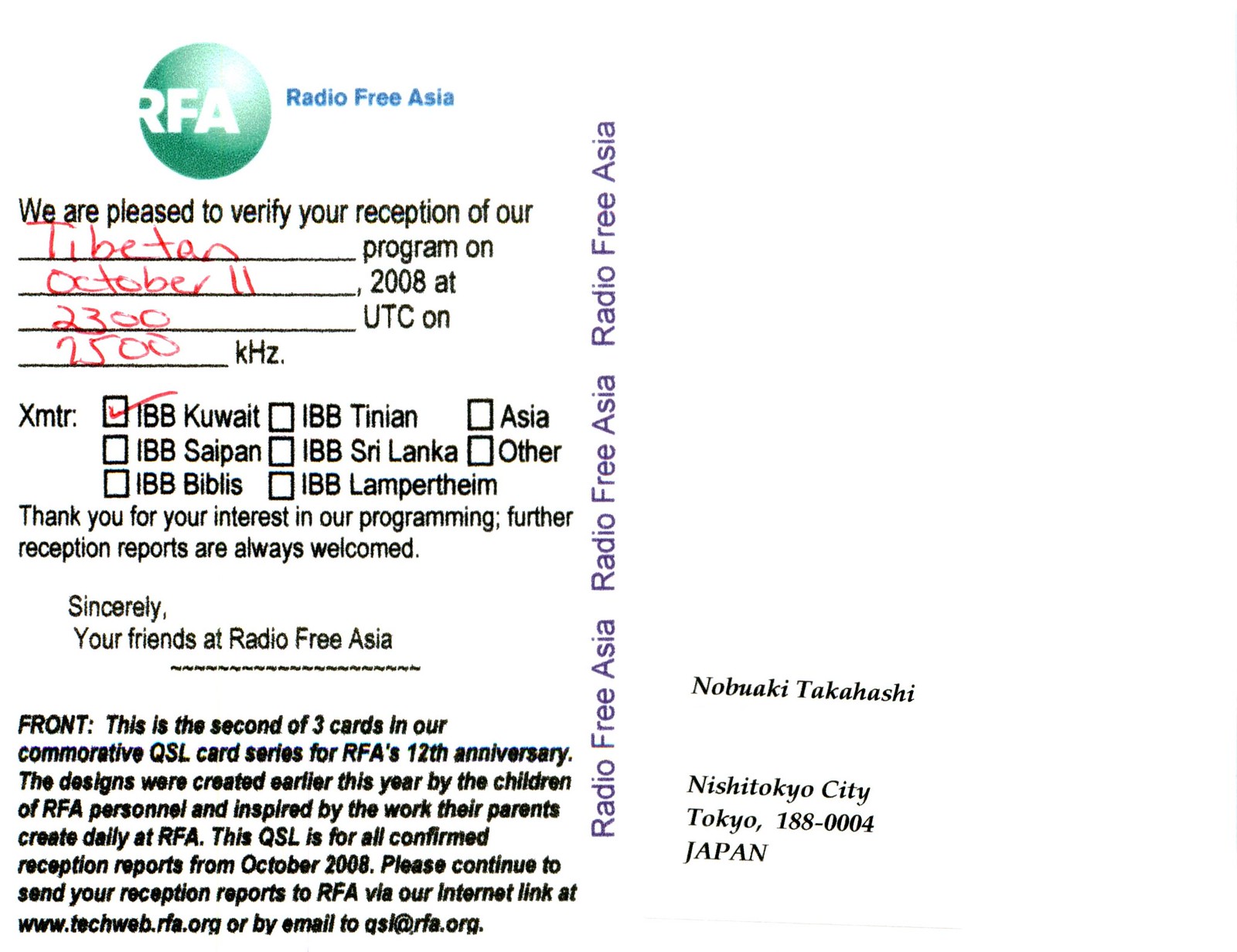This image depicts a landscape-oriented, printed postcard from Radio Free Asia, primarily designed for ham radio operators to confirm signal reception. The card features a color logo on the top left with a green circle and white "RFA" lettering inside, accompanied by "Radio Free Asia" in blue text to the right. Vertically, "Radio Free Asia" is repeated three times in purple for header consistency.

The central section includes a verification statement: "We are pleased to verify your reception of our Tibetan program on October 11, 2008, at 2300 UTC on 7500 kHz, XMTR IBB Kuwait," with this specific information filled in by hand in red ink. Below this, there are several checkboxes listing locations such as Saipan, Byblos, Lamprotheim, Sri Lanka, Tinian, Asia, and Others; only "IBB Kuwait" is checked.

A friendly note reads, "Thank you for your interest in our programming. Further reception reports are always welcomed. Sincerely, your friends at Radio Free Asia." The right section of the postcard is addressed to Nobuaki Takahashi, Nishitokyo City, Tokyo, 111-888-0004, Japan.

A commemorative disclaimer notes this as the second of three QSL (verification of reception) cards celebrating RFA’s 12th anniversary. It highlights that the designs were created earlier that year by the children of RFA personnel, inspired by their parents' work. The lower left corner provides additional contact information advising recipients to send further reception reports via the internet at www.techweb.rfa.org or by email to asi@rfa.org.